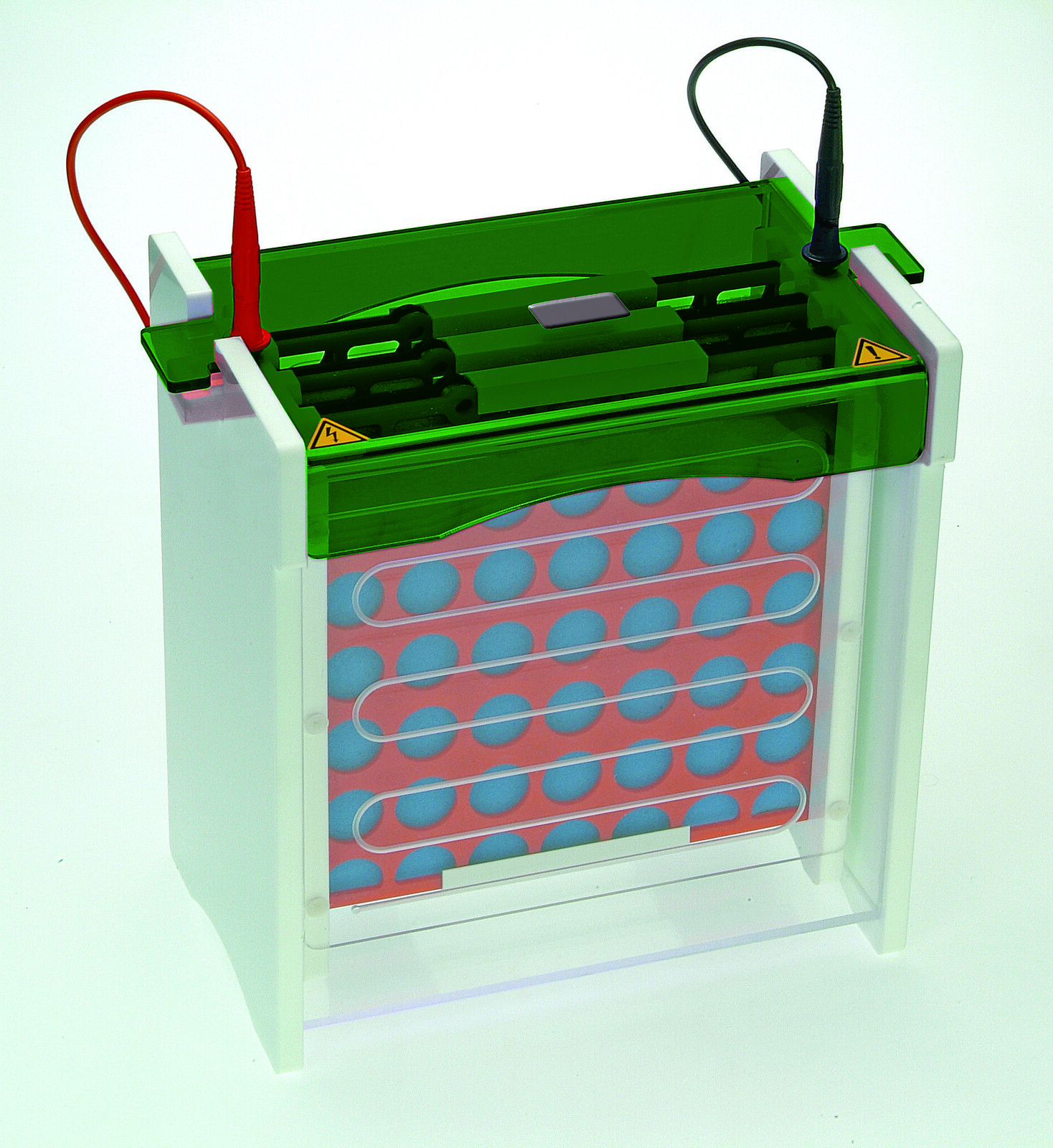This digital illustration, rectangular in shape, predominantly features a machine set against a very light green background. The focal point of the image is a piece of equipment that is similar in appearance to a Connect 4 game, with a structure in the front resembling a filter covered with blue circles on a red background. The unit, which evokes the look of a printer, has three slots on top designed for filters. Tubing extends along the top, implying some functionality related to fluid or air movement, and there are wires attached to both sides—one black and one unidentified color—plugging into the top, each next to a yellow warning sticker. The illustration lacks explanatory text, suggesting it is meant for an instruction manual. Additionally, the left and right sides of the machine have features that bring to mind car jumper cables, hinting at its potential use in electrical or automotive applications. This graphic-made illustration emphasizes the electronic and mechanical aspects of the equipment, showcased through its design and associated warning indicators.